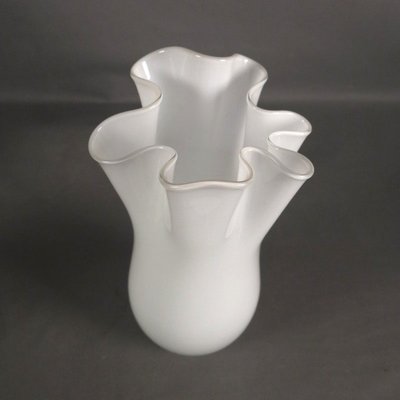The image depicts a white, glass vase with a unique, scalloped top that resembles the irregular shape of a partially open sack or plastic bag. The vase sits on a gray surface with a simple, gray background that shows subtle variations in tone. A faint line in the background suggests the division between a floor and a wall. The vase features a rounded bottom and a silver band around its wavy rim, adding a slight touch of contrast to its otherwise plain, white design. The overall scene is minimalistic, focusing solely on displaying the vase without any additional elements or distractions.